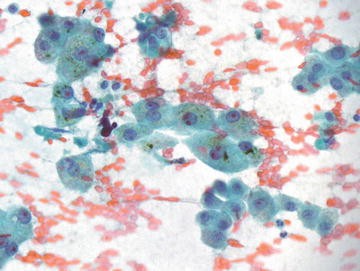The image presents a detailed and intricate view akin to what one might see under a microscope in a biology class. It features a predominantly white background, punctuated by clusters of reddish-pink and teal-blue circular shapes. The reddish-pink circles are small, numerous, and gathered into various clusters, possibly depicting blood cells or similar biological structures, numbering around a hundred. Interspersed among these are larger teal circles, each containing a darker blue center, with approximately fourteen of these aggregate structures scattered throughout the image. Adding to the complexity is a small black area located in the left third of the picture, enhancing the abstract and organized chaos of the scene. The juxtaposition of the red and teal hues on a stark white backdrop creates a compelling, almost watercolor-style artwork that blurs the line between scientific imagery and abstract art.